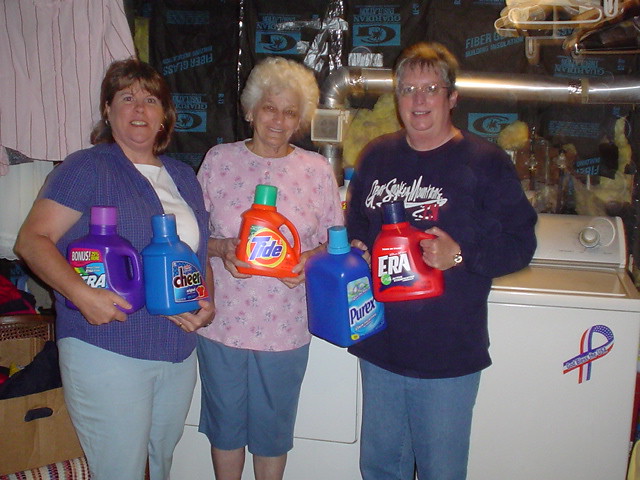In this detailed photograph, three women, possibly from the same family, are standing in a cluttered laundry room and holding various bottles of liquid laundry detergent while smiling at the camera. The woman on the right, dressed in a long-sleeved purple sweatshirt adorned with unreadable white text and jeans, holds bottles of Aera and Purex laundry soap. The woman in the middle, appearing to be the oldest and likely the grandmother, sports a pink floral-patterned top and a denim skirt while clutching a bottle of Tide detergent. The woman on the left, in a blue top and light blue pants with shoulder-length brown hair, balances bottles of Cheer and Extra laundry soap. The background reveals piles of insulation tacked to the walls, a washer, and a dryer, with the latter decorated with a red, white, and blue ribbon sticker that says "God Bless the USA." A dryer vent can be seen extending to the right, while a shirt hangs on the left, completing the domestic scene.